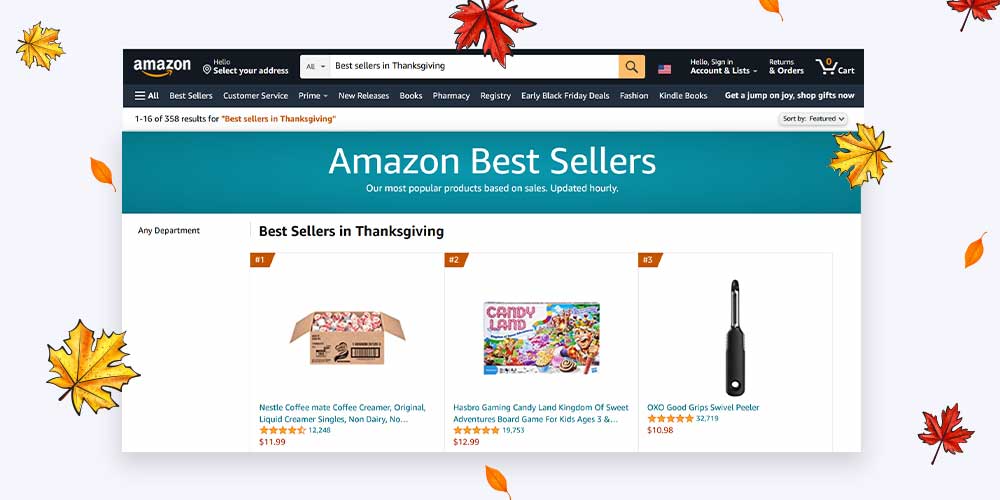The image is a screen capture of the Amazon shopping website, displayed on a very light pastel lilac background. This lilac background is adorned with autumn leaves in vibrant shades of gold and red. The Amazon webpage itself features a white background. At the top of the page is a green horizontal banner, overlaid with white text that reads, "Amazon Best Sellers." Below this, in smaller text, it states, "Our most popular products based on sales updated hourly." Just beneath this green frame, there is another black frame. Further down on the white background, bold black text announces the section: "Best Sellers in Thanksgiving."